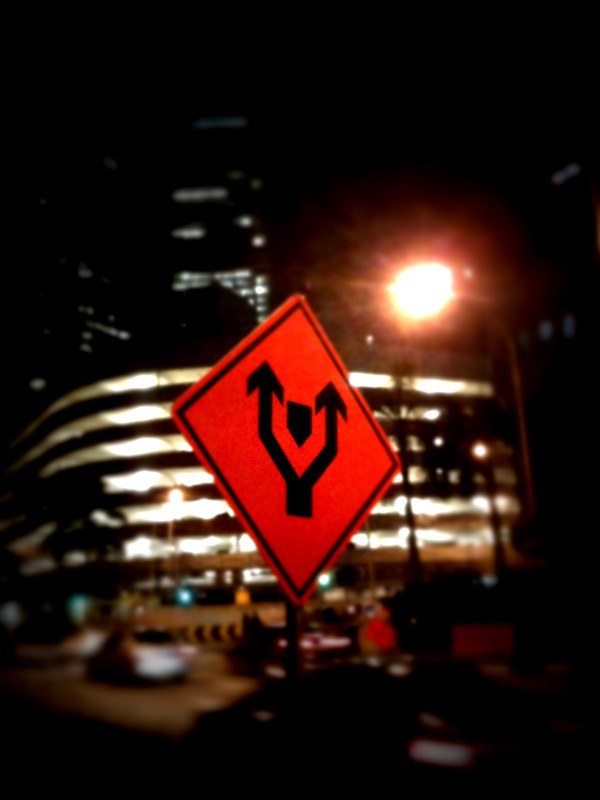This nighttime photograph features a centrally placed orange street sign with a black border. The sign displays two split black arrows pointing upward, with a shield-shaped black symbol in the center. In the background, a large building is softly illuminated with white light, standing in front of a skyscraper that also glows with a similar soft white hue. To the side of the image, an amber-glowing street light adds warmth to the scene. Near the bottom, several cars are visible, including a lighter-colored one, along with concrete barriers. Additionally, a black and yellow striped object and a green traffic light can be seen, adding more elements to this urban nightscape.